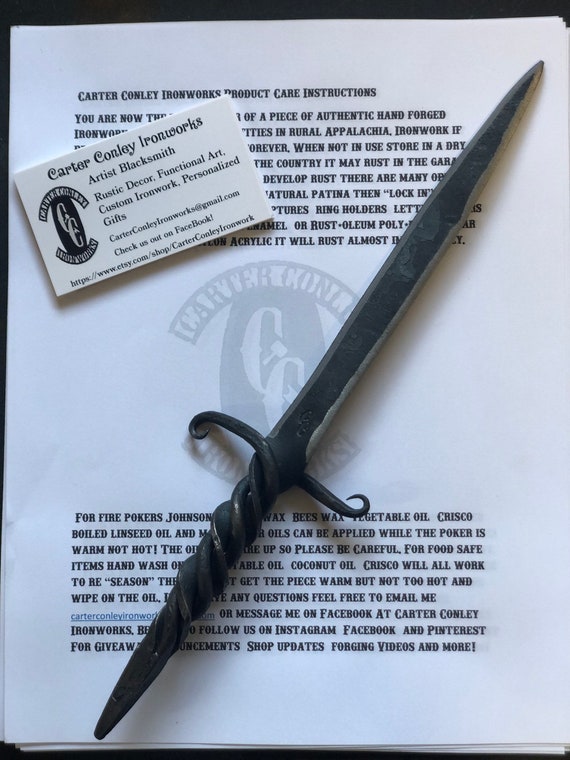The image displays a hand-forged, wrought iron dagger with a dark, blackish-gray hue. The double-sided blade, approximately 12 inches in length, transitions into a handle crafted from the same metal, intricately twisted into a helix-like spiral. The guard at the top of the handle features two inwardly curled spikes, adding to its rustic and artistic design. The dagger rests on a piece of paper titled "Carter Connelly Ironworks Product Care Instructions," which provides guidelines on maintaining the dagger using various oils and waxes when slightly warm. Partially covering this paper is a business card for Carter Connelly Ironworks, promoting their services in artist blacksmithing, rustic decor, functional art, custom ironwork, and personalized gifts. The card includes contact information and social media links, emphasizing the authenticity and handcrafted nature of the ironwork.